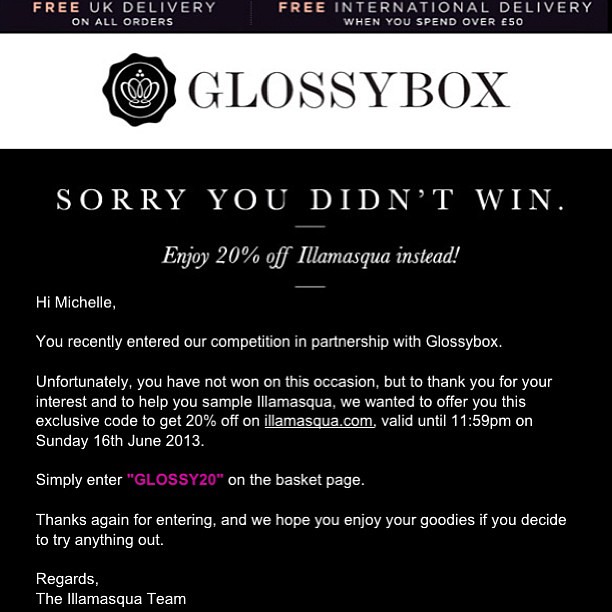The image is a black and white advertisement for Glossybox with a simple and clean design. At the top, a black border features the text: "Free UK delivery on all orders," on the left, and "Free international delivery when you spend over £50," on the right. Below this, a white banner displays the Glossybox logo, a tiny crown encircled, accompanied by the company name in bold black capital letters. The main section of the image consists of a solid black background with white text. At the top of this section, bolded text reads, "Sorry you didn't win." Underneath, it offers, "Enjoy 20% off La Moskva instead." The message continues in a left-aligned format: 

"Hi Michelle, you recently entered our competition in partnership with Glossybox. Unfortunately, you have not won on this occasion, but thank you for your interest. To help you sample La Moskva, we wanted to offer you this exclusive code to get 20% off on our website. This offer is valid until 11:59 PM on Sunday, the 16th of June. Simply enter 'Glossy20' in the basket page."

The exclusive code, "Glossy20," is prominently displayed in purple text. The message concludes with a thank you for entering and hopes that Michelle enjoys her goodies if she decides to try anything out. The overall presentation suggests that the message is either from an online advertisement or a digital image, designed to catch the reader's attention with its striking contrast and clear information.